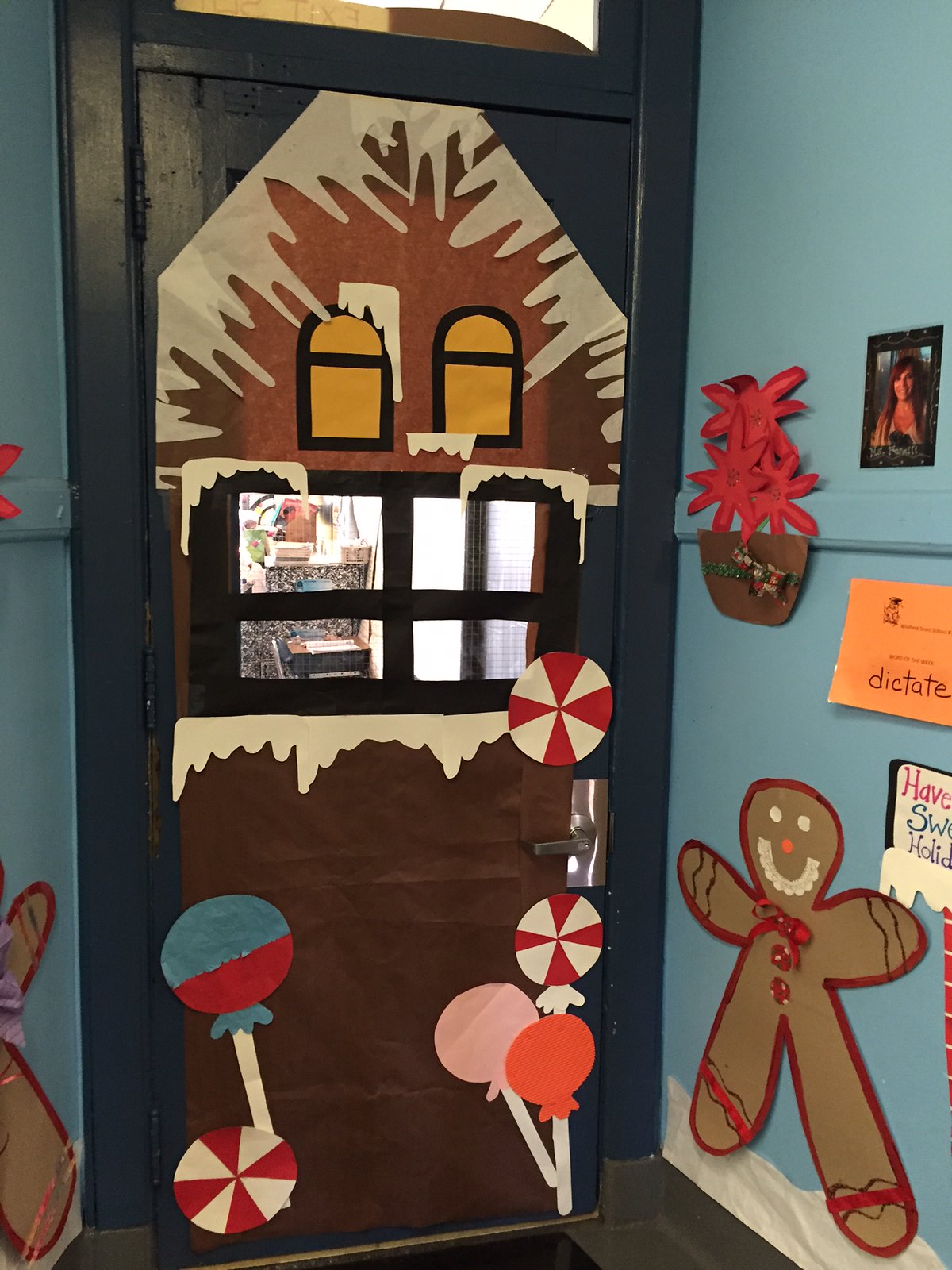The photograph captures a festively decorated door, likely located in a school or daycare setting, adorned to resemble a gingerbread house for the Christmas season. The door itself is a steely dark blue, framed by light sky-blue walls. The upper and lower sections of the door are plastered with brown paper to suggest the gingerbread base, while meticulously trimmed white paper mimics snow and icicles draping from the roofline.

Central to the door is a faux window made from black construction paper, featuring four window panes that provide a peek into an adjacent room's shelving and desk setup. Flanking the window, yellow paper forms two additional mock windows with a black rectangular base, topped with more white paper simulating snowy eaves.

Decorative peppermint and lollipop designs are strategically placed around the door. A blue and red lollipop and a peppermint candy sit on the left, while a red and white peppermint and an orange and pink lollipop embellish the right side beneath the silver door handle.

The surrounding wall features further festive touches, notably a gingerbread man outlined in red with white eyes, a mouth, and a pinkish-red nose. Above him is an orange sign, partially visible, which likely reads "Have a Sweet Holiday," accented by the word “dictate” in lower script. Adjacent to this, a photograph of a young woman—possibly a teacher named Mrs. Finnelli—adds a personal touch. Completing the scene is a vibrant construction paper poinsettia decoration with three red flowers in a brown pot, positioned to the left of the photo.